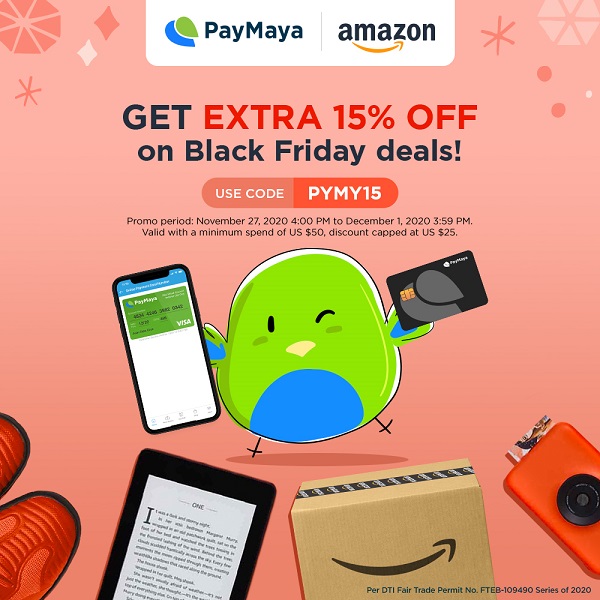**Image Caption:**

The display ad is a square-shaped graphic with a vibrant pink background. At the top, a horizontally oriented rectangle with rounded corners is divided between two logos. On the right side, the Amazon logo appears in black lowercase letters, featuring the distinctive gold arrow resembling a smile. On the opposite side, the logo for PayMaya is displayed, with "PayMaya" written in black font and characterized by the capital letters "P-A-Y-M-A-Y-A" joined together. Adjacent to the text, the PayMaya logo includes two inverted teardrops, one blue and the other olive green.

Centered on the pink background, the primary promotional text reads "Get Extra 15% Off on Black Friday Deals." The "Extra 15% Off" portion stands out in bold red capital letters, while the rest of the message is in black font.

Beneath the promotional text, another rounded rectangle displays a discount code. On the left side of this rectangle, white text on a pink background instructs to "Use Code." On the right side, against a red background, the discount code "PYMY15" is prominently presented in white uppercase letters.

Lower in the ad, a green cartoon character resembling a jelly bean appears, potentially serving as a company mascot. This character, which might be a bird, is depicted with minimalistic lines for eyes and a small beak. One wing holds a smartphone, while the other grasps a credit card, hinting at the company's involvement in payment services.

Finally, at the bottom of the square, a brown cardboard box featuring the Amazon smile logo is positioned alongside a Kindle e-reader, open to an indiscernible page from a book.